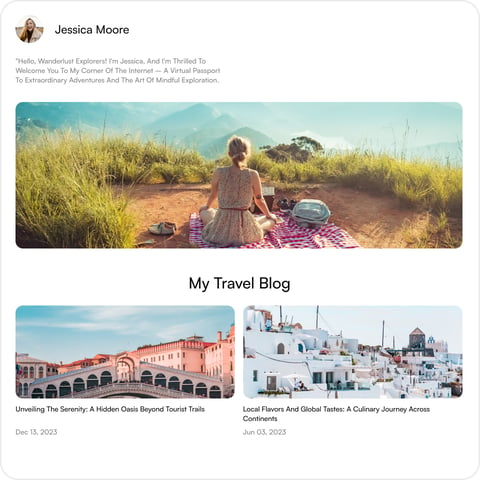A blog by Jessica Moore features a prominent profile picture of Jessica, a fair-skinned woman, located at the top left of the webpage. Beside her image is a welcoming message: "Hello wanderlust explorers, I'm Jessica and I'm thrilled to welcome you to my corner of the internet, a virtual passport to extraordinary adventures in art and the art of a mindful exploration." 

At the top of the page, a wide image features Jessica at the summit of a mountain or hill, sitting on a picnic blanket in a cross-legged, meditative posture. She is wearing a sundress, facing away from the camera, and gazing into the distance, evoking a sense of peaceful contemplation.

Beneath this, there are two additional photographs, each accompanied by its own description. The first image shows an old village reminiscent of Italy, titled "Unveiling the Serenity: A Hidden Oasis Beyond the Tourist Trails." The second photograph depicts a scene reminiscent of Greece, titled "Local Flavors and Global Tastes: A Culinary Journey Across Continents." Both posts were published in 2023. The blog appears to be a general exploration of diverse destinations and experiences without focusing on a specific location.